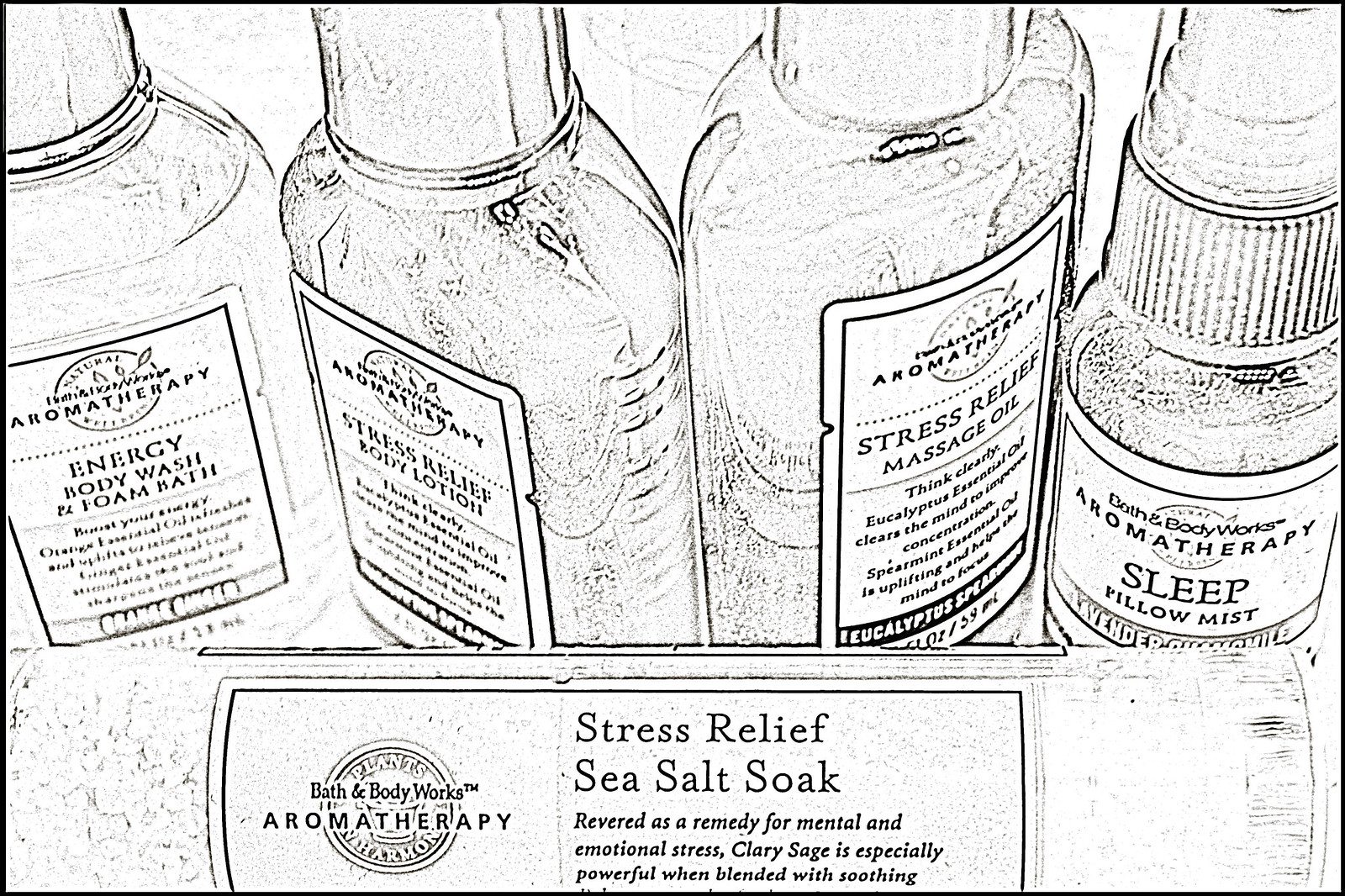This detailed, black-and-white sketch features a close-up array of Bath & Body Works aromatherapy products. In the forefront lies a horizontal cylindrical bottle labelled "Aromatherapy Stress Relief Sea Salt Soak," noted for its powerful blend of Clary Sage, revered as a remedy for mental and emotional stress. The background showcases four upright bottles: from left to right, they are "Emerge Energy Body Wash and Foam Bath," "Stress Relief Body Lotion," "Stress Relief Massage Oil," and "Aromatherapy Sleep Pillow Mist." Rendered with intricate black lines against a stark white backdrop, the image resembles a charcoal drawing or an embossed photograph, emphasizing the contours and labels of each product.